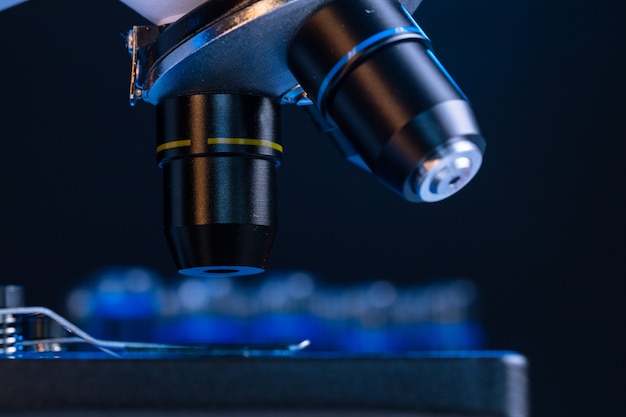The image showcases a close-up view of the imaging end of a white microscope against a black background. The focal point is a rotating lens plate in silver, holding at least two, possibly three, black lens assemblies. These lenses, essential for imaging, have color-coded trims with one in blue and the other in yellow, and they are also accented with gold and silver trims. The lenses are positioned such that one is pointing down towards where the sample would be placed, while the other sticks out. Below the lens assemblies, there is a space of approximately an inch leading to the microscope's stage, which includes a silver clip to secure slides. This detailed and concentrated view only highlights these specific parts of the microscope, leaving the rest of its structure indistinct.